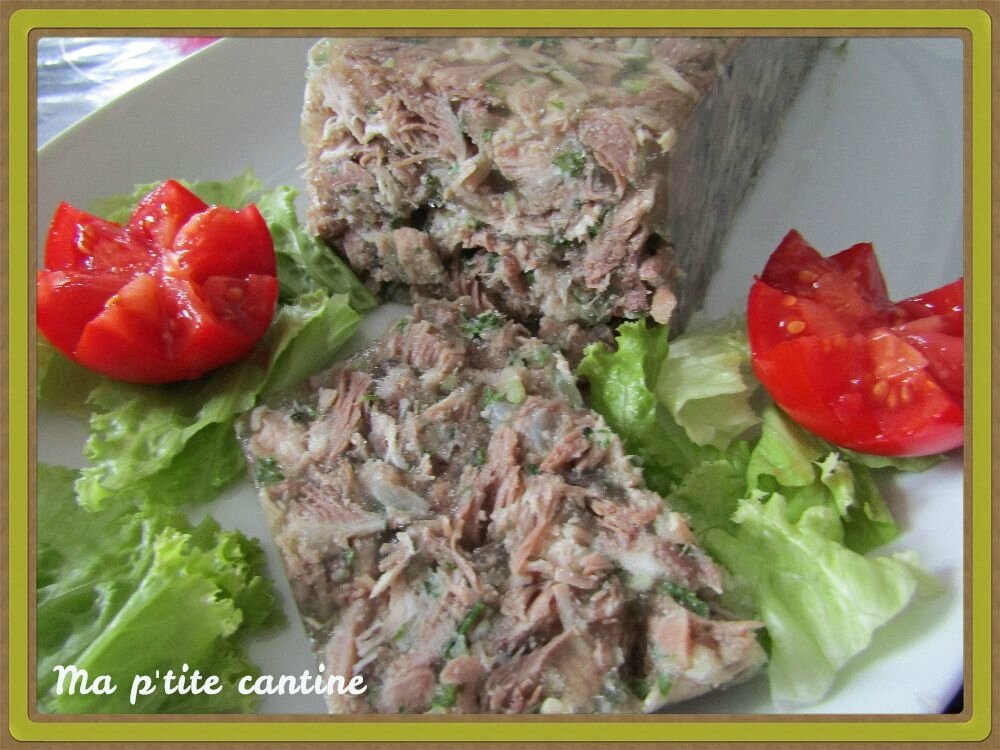In the center of the image is a rectangular block of light brown pulled meat mixed with a gelatinous substance and green vegetables, encased in a clear gel. The pulled meat is displayed on a large, oval white plate. On both sides of the meat block are half-cut tomatoes intricately sliced into triangular, star-like shapes, with visible seeds. Pieces of fresh lettuce are arranged around the front of the plate. The background includes a brown border with a yellow square in the middle, and the bottom left corner of the image features white text spelling out "M-A-P-T-I-T-E-C-A-N-T-I-N-E." This detailed arrangement suggests a presentation in a restaurant or a kitchen setting.